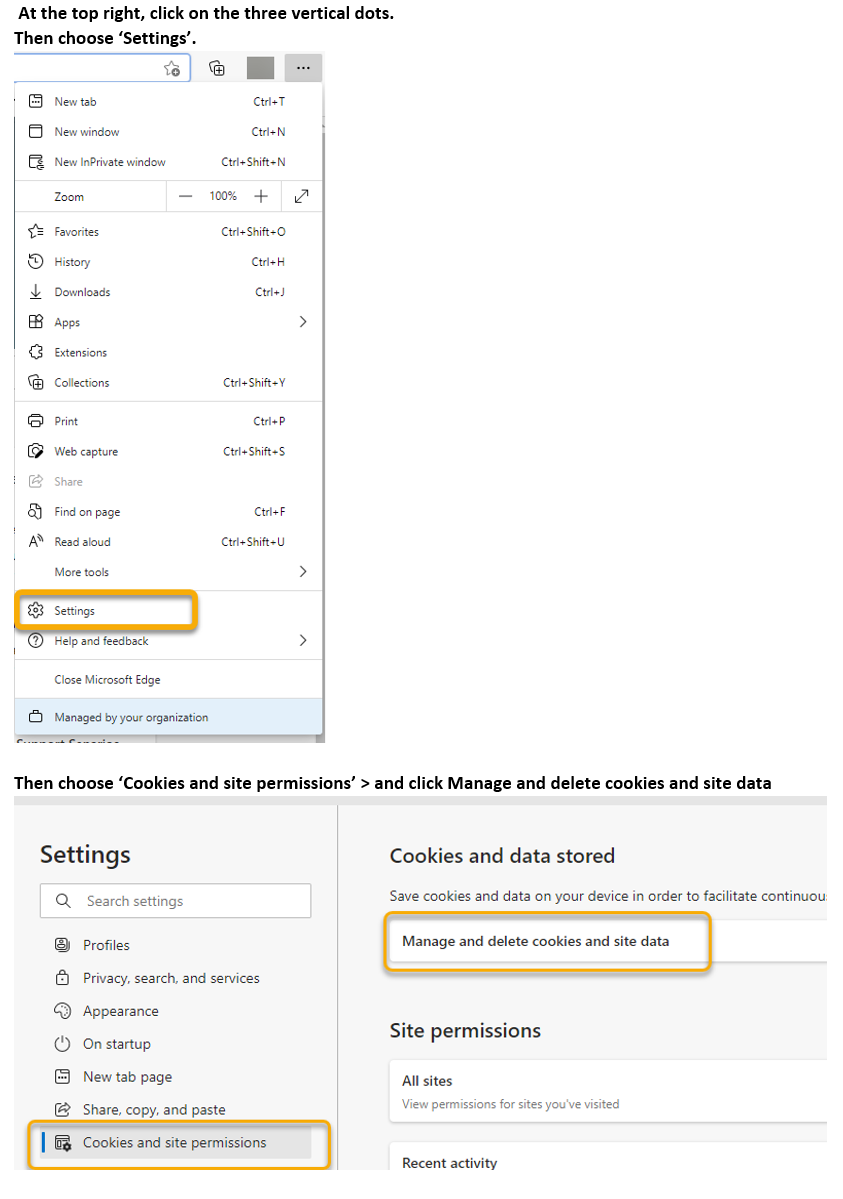The composite image features two distinct sections: a vertical image on top and a horizontal one below it.

In the vertical image, positioned at the top right, is a prompt instructing the viewer to "click on the three vertical dots, then choose Settings." Beneath this text is a blue-outlined rectangle, which contains a star icon and a gray dot in its bottom right corner. Adjacent to this are two stacked boxes. Below these boxes is a solid gray box, followed by another gray box containing three horizontal dots. To the right of these elements is an icon designated for opening a new tab, with the command "Ctrl + T" displayed next to it. Further right, there is an icon for opening a new window with the command "Ctrl + N" indicated beside it. Additionally, there's an icon for initiating a new private window, accompanied by the command "Ctrl + Shift + N."

The horizontal image extends below, showcasing three distinct rectangular boxes in sequence. The first box is labeled "Zoom," followed by another box marked with a plus and minus sign, "+ 100 -". An arrow within this box points diagonally from the upper right to the lower left. The final rectangular box features a star icon accompanied by three lines and includes the label "Favorites," along with the command "Ctrl + Shift + O."